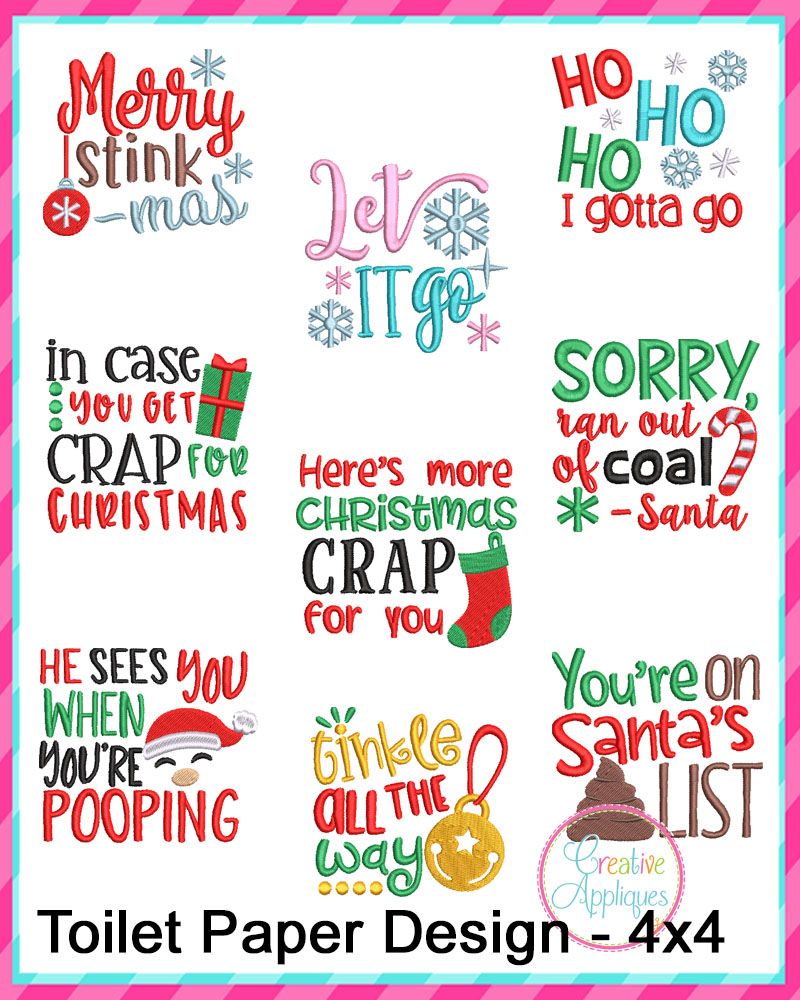The image shows a colorful advertisement for Creative Appliques' toilet paper designs, framed with light pink and dark pink candy cane stripes, and bordered further with thin turquoise blue and light turquoise blue stripes. At the bottom, it reads "Toilet Paper Design 4x4" and features various Christmas-themed designs, each with distinctive typefaces and colors. 

The playful holiday phrases include "Merry Stinkmas" with 'Merry' in red cursive, 'Stink' in brown, and 'Dashmas' in blue, accompanied by snowflakes and an ornament. Another design says "Let It Go" in pink and turquoise with additional snowflakes. The humorous "Ho Ho Ho, I Gotta Go" also features snowflakes, while "Sorry, We're Out of Coal, Santa" includes a candy cane and green snowflake. 

Other designs are "Here's More Christmas Crap For You" with a stocking, and "In Case You Get Crap for Christmas" with a green and red present. "He Sees You When You're Pooping" showcases a Santa face graphic, "Tinkle All The Way" has a bell with a red string, and "You're On Santa's Poop List" humorously highlights a cartoon pile of poop. The Creative Appliques logo is prominently displayed at the bottom right of the advertisement.